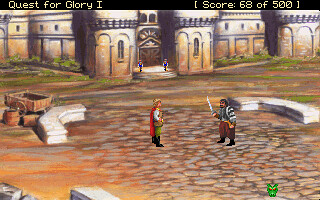This image is a square-shaped screenshot from a gameplay scene of "Quest for Glory I." At the top left corner, the game title "Quest for Glory I" is prominently displayed, and at the top right, the score is shown as "[Score: 680/500]" in a yellow font. The background features a strip of black, adding contrast to the scene.

In the forefront, centrally positioned, there are two characters: one in a more prominent middle position and another to the right. Additionally, two more characters are present in the far background. The setting includes an imposing castle with a prominent brown door, flanked on either side by sentinels or guards standing watch. The combination of characters and the intricate castle details enhance the immersive fantasy atmosphere of the game.